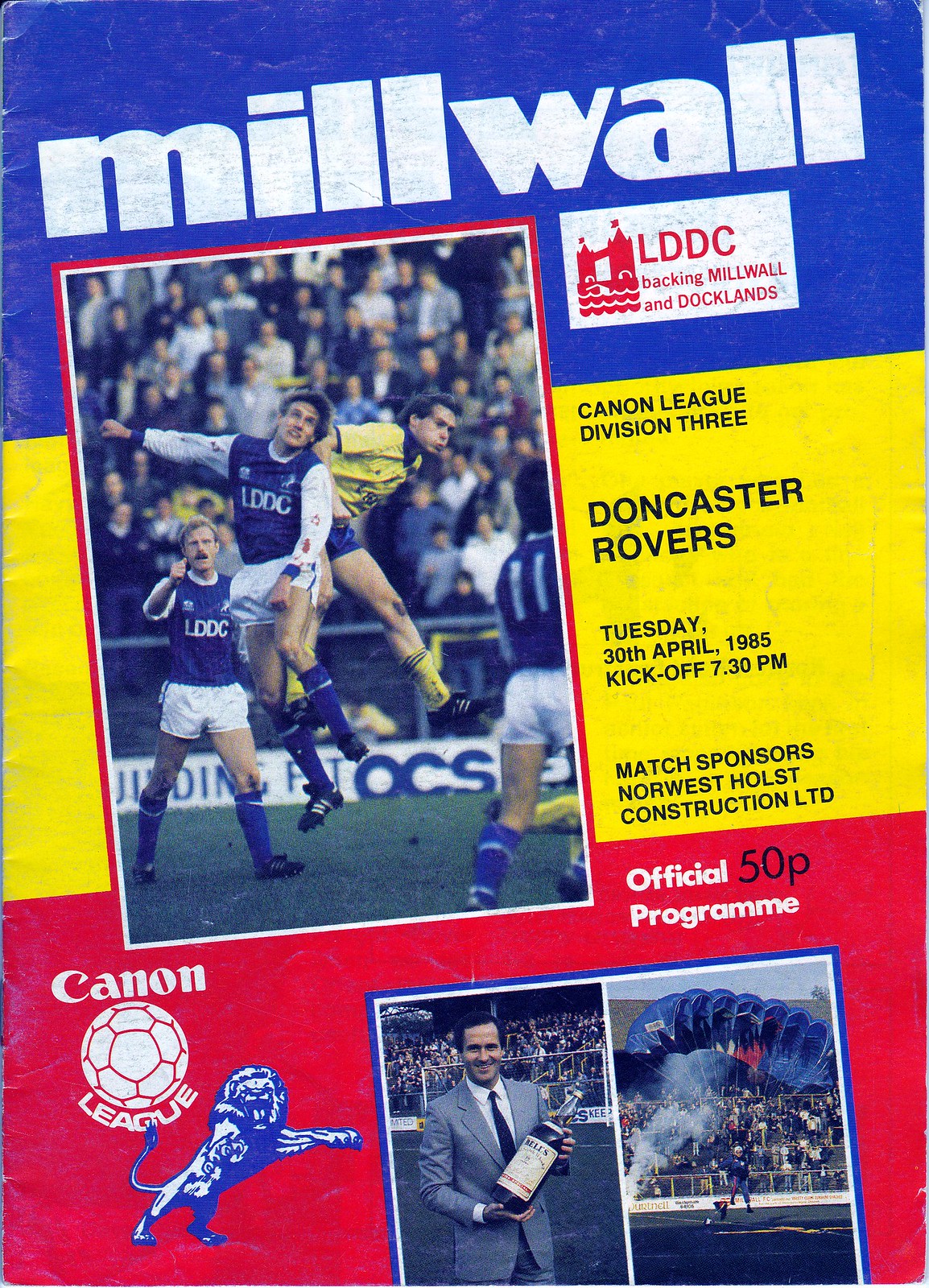This vintage poster, dating back to April 30, 1985, serves as an official program for a Millwall soccer match in the Cannon League Division III against Doncaster Rovers, with a kickoff time of 7:30 p.m. The design features three main colors: blue at the top, yellow in the center, and red at the bottom. The title "Millwall" is prominently displayed in large white text across the top blue section. The central part of the poster contains a photograph capturing two soccer players in mid-air, donning blue shirts with "LDDC" on the front and white shorts, seemingly jumping towards a soccer ball. Additional details include a listing of the match sponsors, Northwest Holst Construction, LTD, and a note on the price at the bottom red section: "Official Program 50-P." Also featured are images of a man in a suit holding a large bottle of red wine and another individual landing with a parachute in a stadium. The poster encapsulates the excitement and sponsorships of this 1985 soccer event.